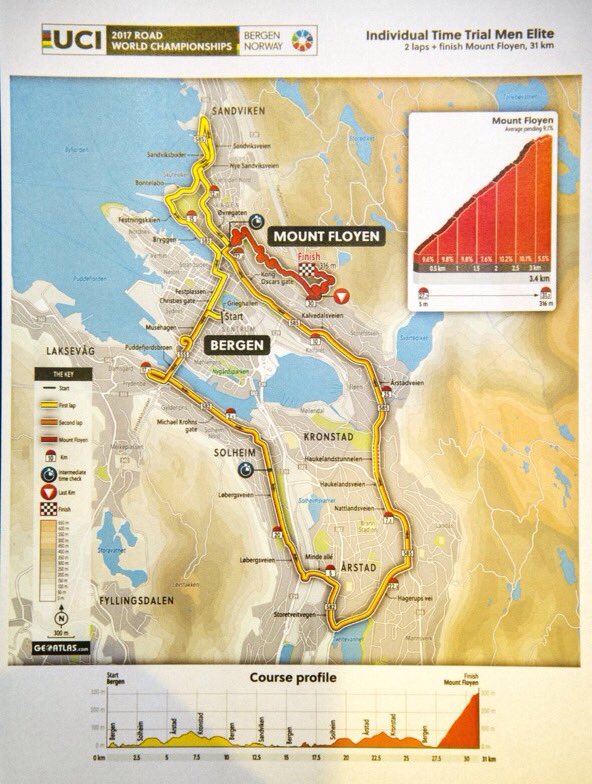This image features a detailed graph set against a white-colored background at the top and bottom. In the top left corner, text reads: "UCI 2017 Road World Championships, Bergen, Norway." Specifically, "Bergen" is spelled B-E-R-G-E-N. To the right, additional text indicates, "Individual Time Trial, Men Elite, Two laps, Finish Mount Fløyen," with "Fløyen" spelled F-L-O-Y-E-N, and the distance specified as 31 km.

Central to the image is the graph itself, displaying a prominent yellow line that indicates a particular trajectory or trend. Above this yellow line is a smaller red line. The top of the graph is labeled "Mount Fløyen."

To the right of the line graph, there is a bar graph that extends vertically, featuring bars colored in red and orange hues. The top of this section is also labeled "Mount Fløyen."

Additionally, towards the bottom left of the image, there is a section with a labeling icon, which might provide further details or legends pertinent to understanding the data presented in the graph.